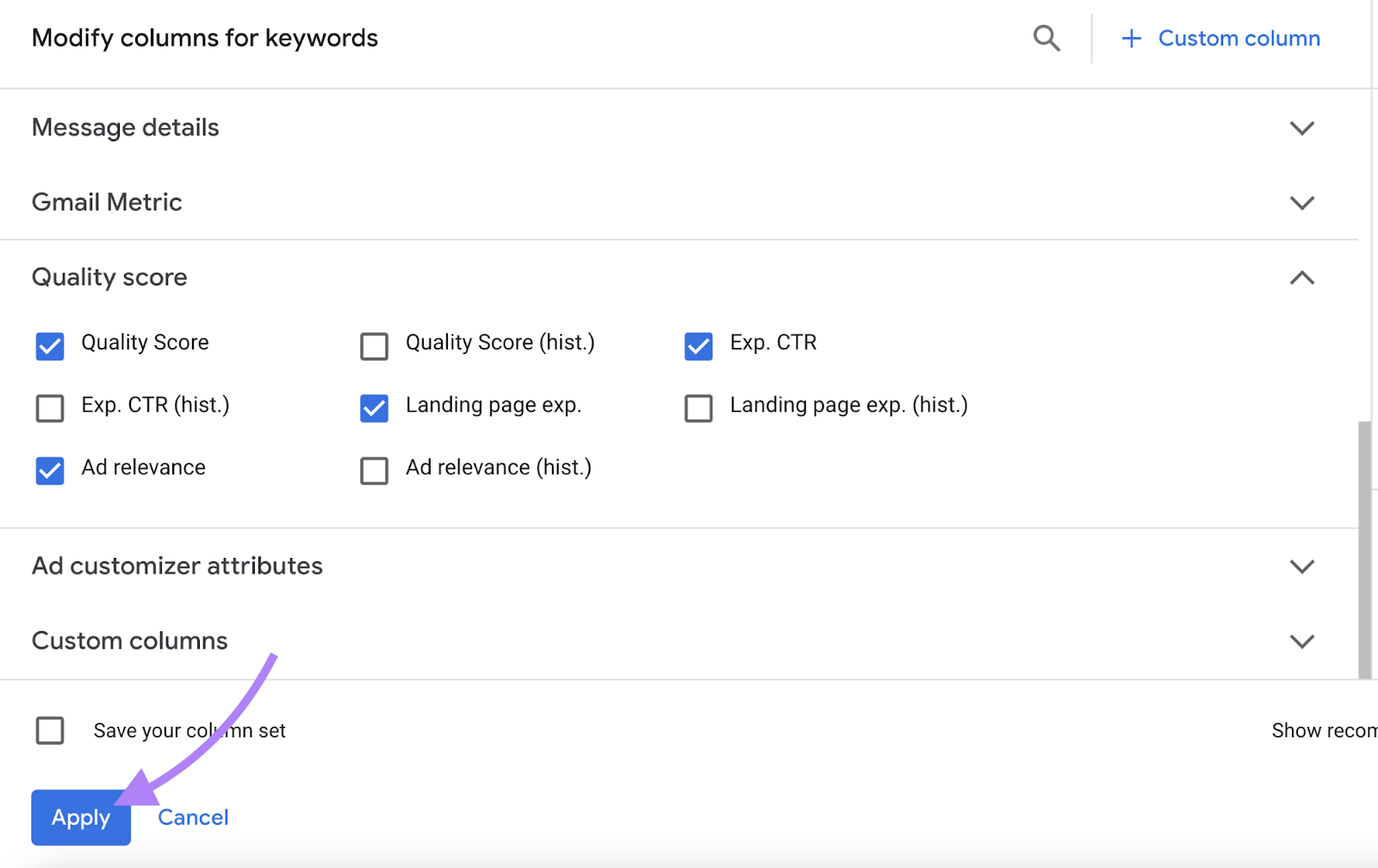This screen capture displays a computer application interface in landscape mode, featuring a predominantly white background with black text. The interface includes several checkboxes, some of which are marked with a blue highlight and a white checkmark. In the upper right corner, there is a blue "Add Custom Column" option. At the bottom left corner of the screen, blue "Apply" and "Cancel" buttons are visible, with a downward-angled lavender arrow pointing towards the "Apply" button. The arrow originates from the top right and curves slightly downwards to the left, directing attention to the button.

On the right side, a gray slider bar indicates that the content has been scrolled to the bottom. Text on the screen is left-aligned, and headings read: "Modify Columns for Keywords," "Message Details," "Gmail Metric," and "Quality Score," accompanied by several checkboxes arranged into three columns. The first and second columns contain three checkboxes each, and the third column contains two checkboxes. Below these sections, additional headers for "Add Customizer Attributes" and "Custom Columns" are present.

The detailed layout emphasizes functionality for modifying columns and customizing the application interface, catering to user preferences and settings adjustments.